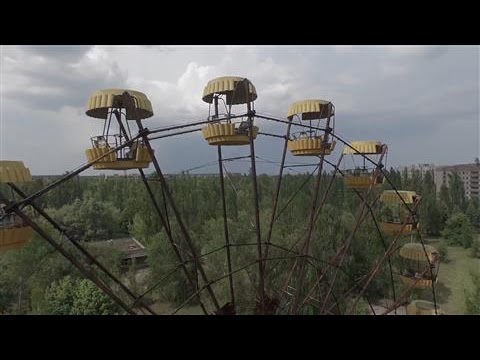This rectangular image, wider than it is tall, framed by black borders on the top and bottom, depicts a dreary, overcast day with a sky almost completely gray and heavy with clouds. Central to the scene is an archaic Ferris wheel, its structure crafted from weathered, brown metal. The Ferris wheel features beige, domed cars with a fluted, scalloped edge, reminiscent of hot air balloon baskets. These cars, likely open in the middle and flanked by metal bars for safety, appear empty, adding to the somber mood of the image. The Ferris wheel is surrounded by a dense cluster of dark green trees and a few gray apartment buildings, contributing to the melancholic, almost cartoon-like ambiance of the scene. The overall aesthetic feels more like a screen capture from a film or animated series rather than a photograph, accentuated by the desaturated, rainy day setting.